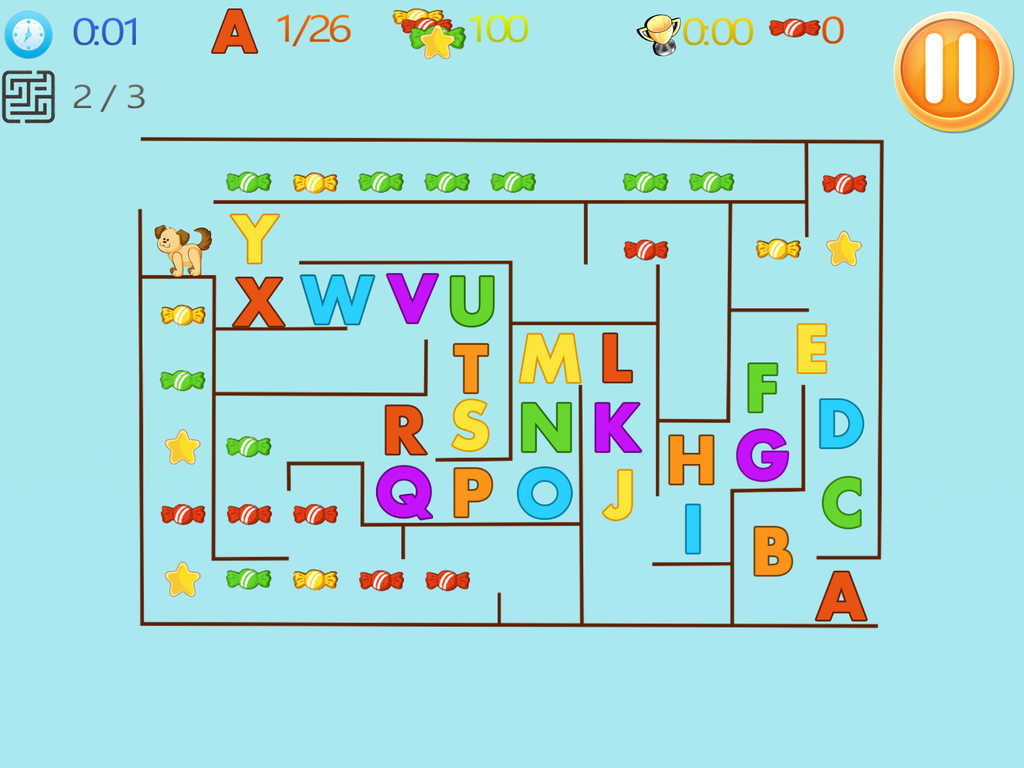Screenshot of an educational game designed for learning the alphabet in sequential order. The entire screen is set against a light blue background. In the upper left-hand corner, there is a timer tracking the duration of play, positioned next to the letter "A" and an indicator showing "1 out of 26" letters learned so far. Adjacent to this, there is a small section displaying candies and stars, with a score of 100 points. Additionally, a trophy icon is showcased next to a secondary timer, alongside another candy icon marked with a zero. A prominent yellow pause button also appears in this area.

Directly below the main timer on the left-hand side, there is an outline of a maze, labeled "2 out of 3." The main section of the page features a simple maze filled with candies in various shades and gold stars, intertwined with alphabet letters. In one corner of the maze, a small dog character is situated, ready to guide players through the learning journey.